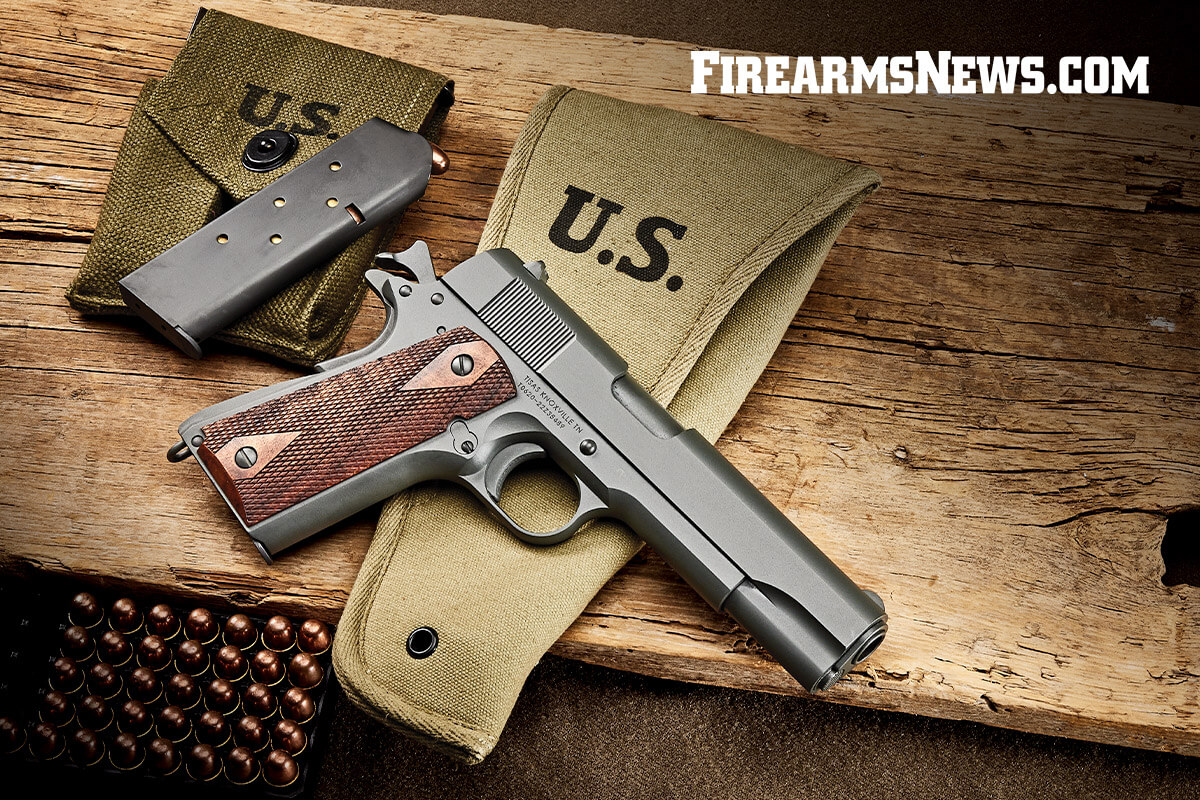The image, taken from firearmsnews.com, features a detailed setup with a prominent large handgun as the focal point. In the top right corner, white capital letters spell out "firearmsnews.com." The gun, a sleek silver pistol with a deep brown handle adorned with small rhombus shapes, is laid out on a plank of weathered wood, showcasing the wood's well-worn grains. Inscribed on the gun are the words "TISSES KNOXVILLE, TN" accompanied by an identification number. The chamber appears to be detached and is resting to the left. Surrounding the gun are army green fabric holsters, each marked with bold black "US" letters. The holsters have buttons and are used to hold the firearm securely. Additionally, a neatly arranged formation of bullets, approximately 30 in total, is visible in the bottom left corner. The entire setup is meticulously arranged, providing a rustic and authentic backdrop for the firearm.